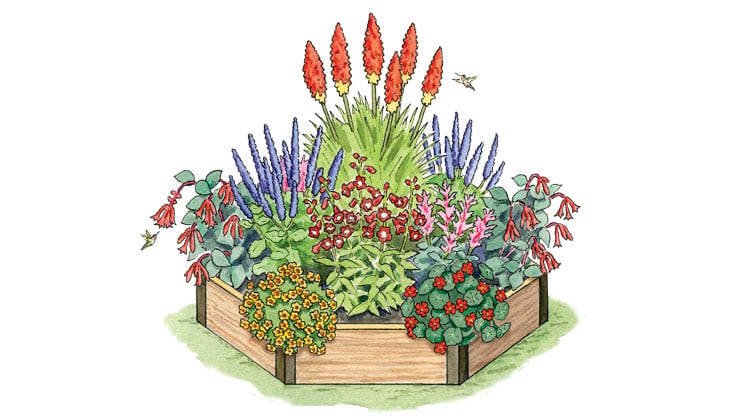The image is a detailed painting of a flower box designed for small yards. The box itself is a six-sectioned, octagonal raised garden made of wood with large timbers at each corner and beige-gray posts around the edges. It's filled to the brim with a variety of blossoming plants against a plain white background. In the center, there is a tall green bush featuring six prominent flame-shaped red blossoms with yellow bottoms that rise high above the other greenery. Flanking the central bush are plants with tall, slender purple blossoms, possibly lavender. There are also flowers on either side that droop down gracefully. Scattered throughout the planter are additional blooms in various shades of red, pink, yellow, blue, and light lavender, contributing to a vibrant, lush display of colors and shapes within the confines of this compact garden.